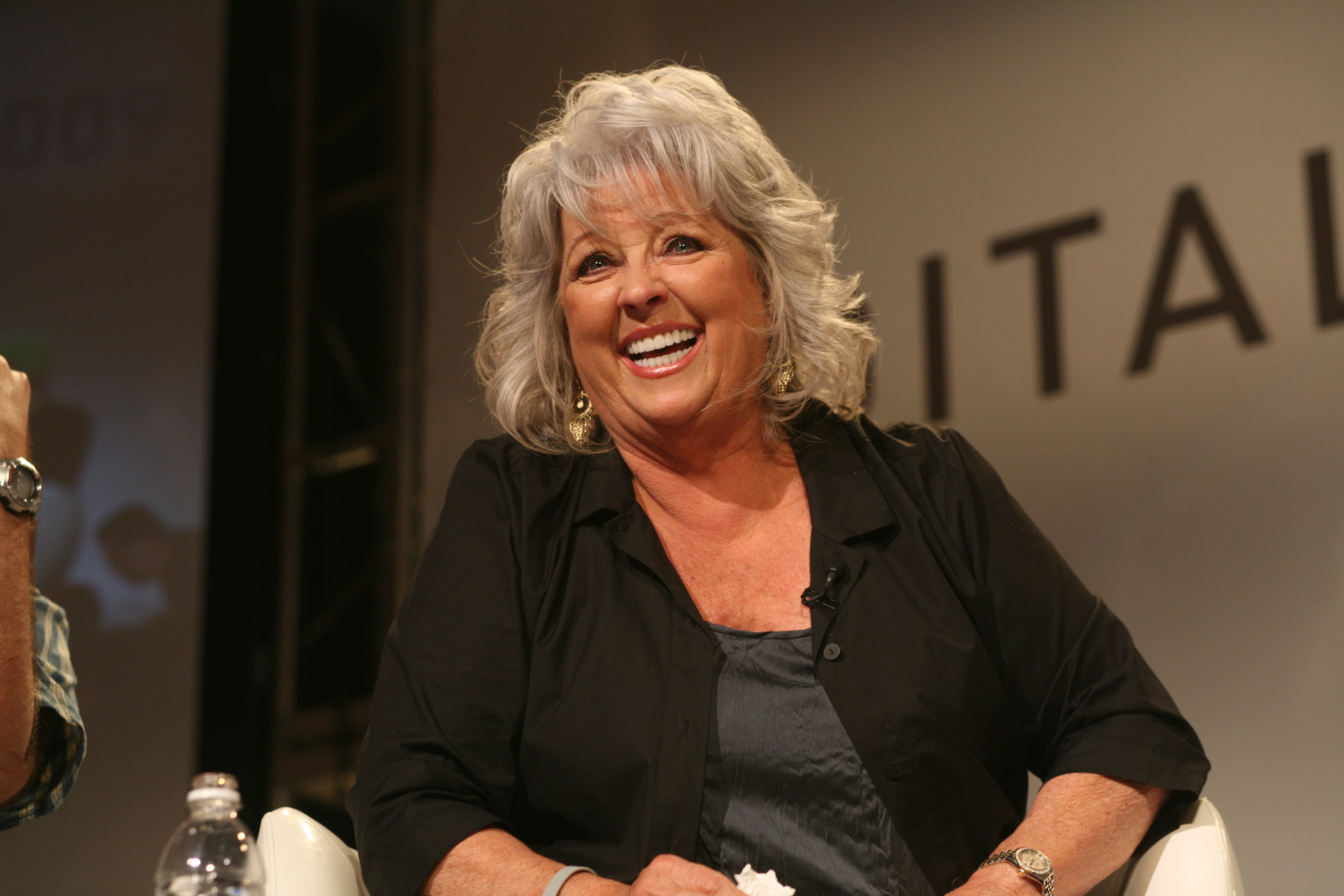The image is a color photograph featuring celebrity chef Paula Deen, captured in what appears to be a TV studio setting, possibly during an interview or meeting. Paula Deen, an older woman with gray-to-white, medium-length wavy hair, is positioned in the center of the frame, sitting in a chair. She is visibly joyous, smiling broadly with her teeth showing, as if she just finished laughing.

Her makeup includes light red lipstick, and she sports a pair of earrings. Paula is dressed in a black button-down shirt with a collar, partially open, revealing a gray tank top or possibly a dark blue shirt underneath. Additionally, she's wearing a watch on her left wrist and has a small black microphone clipped to her shirt.

In the background, letters "I-T-A-I" are partially visible on a white wall, though the complete text is obscured. The colors in the image include shades of black, white, gray, blue, gold, and beige. An arm wearing a watch, presumably belonging to someone else, appears next to her, alongside the top half of a water bottle placed in front of her. The composition suggests a candid moment likely caught by the paparazzi, highlighting Paula Deen's vibrant and cheerful demeanor.